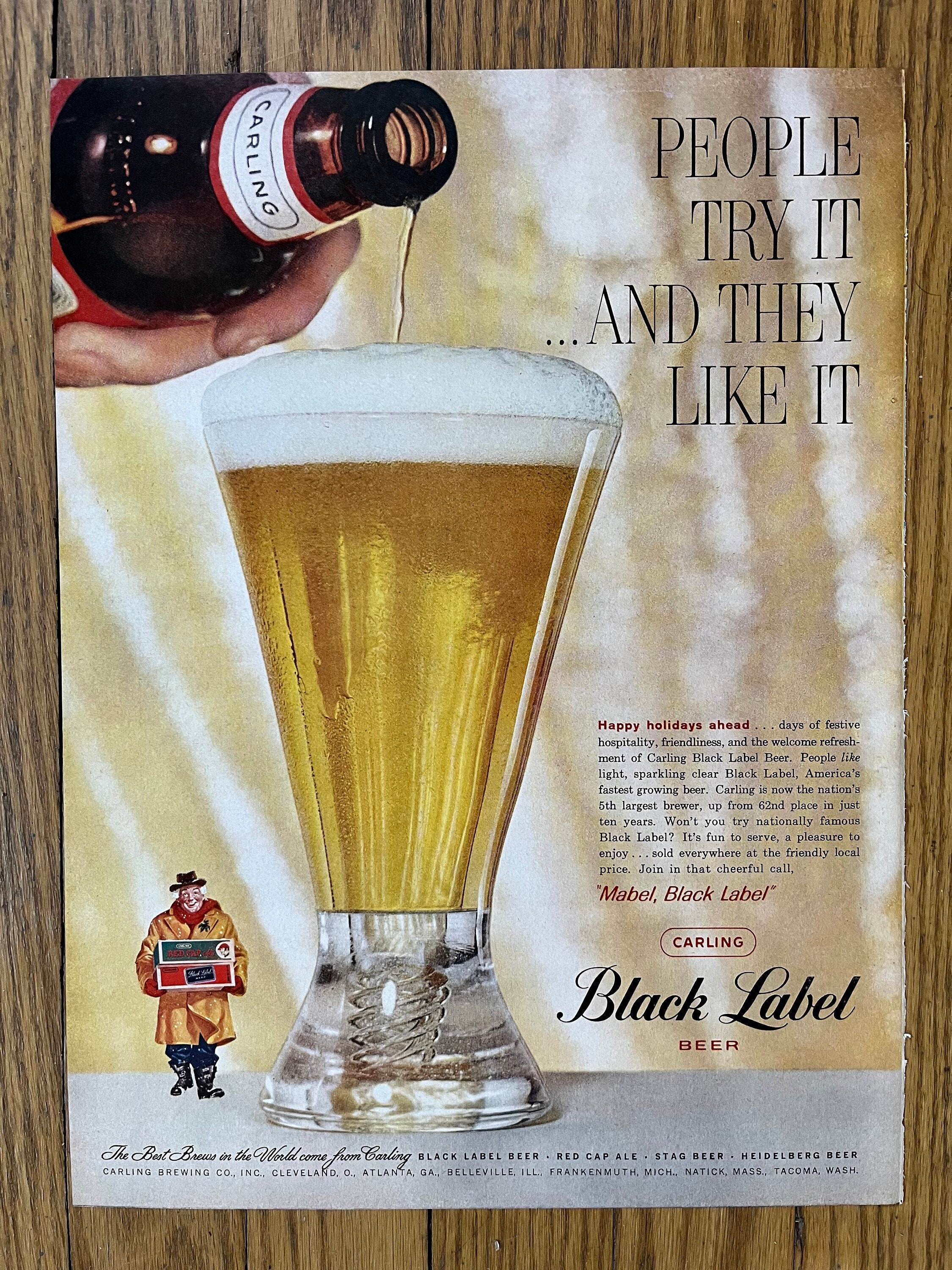The image is a high-resolution photograph of a torn-out page from a magazine, serving as a Carling Black Label Beer advertisement. The rectangular page, roughly 6 inches high by 4 inches wide, is set against a brown wood-paneled background with vertical striations. At the center is a dominant, large glass filled with amber-colored beer crowned with frothy foam, almost overflowing. A dark brown Carling bottle, adorned with a white and red band and marked "Carling" in black print, is seen pouring into the glass. The hand pouring the beer is of Caucasian descent.

In the lower section of the advertisement, there is an illustration of a cheerful man trudging through snow, wearing a heavy coat, black boots, and a hat. He carries two cases of Carling Black Label Beer—one green, one red. The overall scene suggests a festive holiday theme, reinforced by the text "Happy Holidays Ahead" in red, positioned below the man. The top right corner of the ad features the slogan "People try it and they like it" in black print. Below it, in smaller red text, it reads, "Mabel, black label," with further mention of Carling Black Label Beer. A footer at the bottom provides additional promotional information, listing the Carling Brewing Company's various locations across the United States.